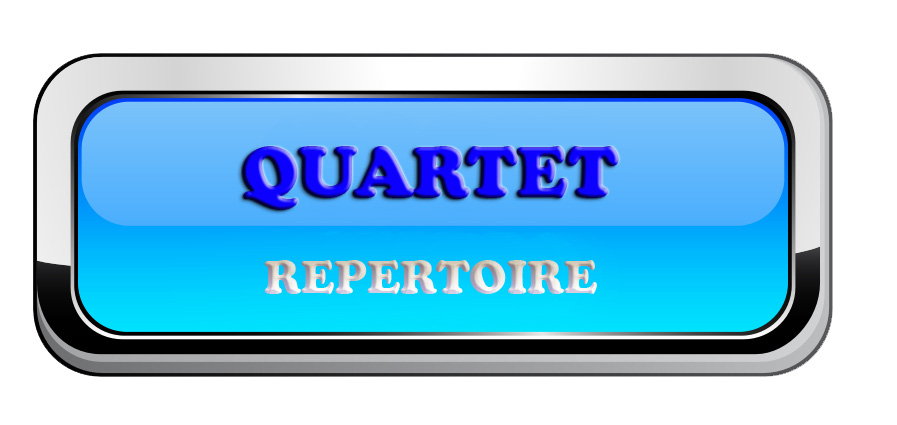The image depicts a horizontal, rounded rectangle with a vibrant blue background. The top portion of the rectangle features a light gray border, while the bottom part has a black border, giving the impression of a reflective or shiny surface. In the center, "QUARTET" is prominently written in dark blue, capital letters, and directly below, "REPERTOIRE" is displayed in white capital letters. The design suggests a clear demarcation between the blues and borders, evoking the look of a license plate or a window pane on a cruise ship, with the blue backdrop reminiscent of a serene ocean or sky on a sunny day.